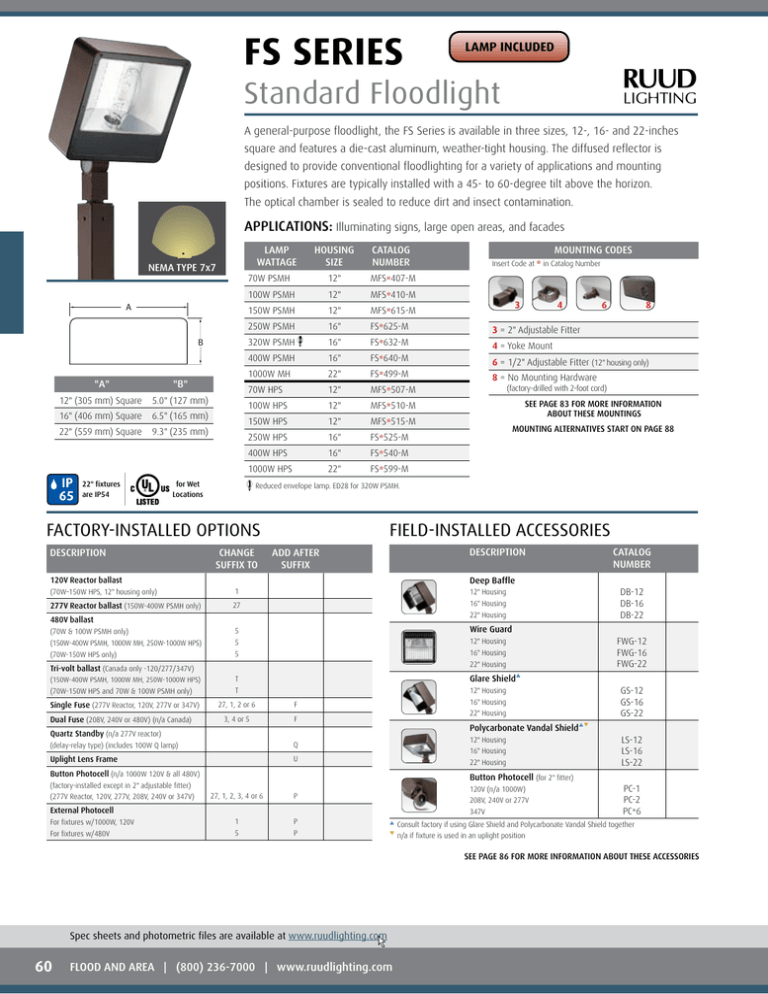This detailed caption provides an intricate description of the image relating to an FS Series standard floodlight by Rood Lighting.

---

The image displays the specifications for the FS Series standard floodlight produced by Rood Lighting, with their name prominently shown in the top right corner in black text. In the upper left corner, there is an image of the floodlight, which is large, rectangular, and emits a bright light. The floodlight has a brown or possibly chromish finish. Below the image, the effective span and radius of the light are detailed. The document contains a total of five tables providing various specifications for the floodlight.

At the top of the document, a paragraph outlines the general purpose of the floodlight, specifying that it is a general-purpose lighting solution available in different sizes: 12", 16", and 22". Additionally, it lists factory-installed options and field-installed accessories.

The document features various colors: black text with shades of grey, white, teal blue, bright cerulean blue, and yellow highlighting the light span description. At the top, there is a notable red text stating "lamp included," which appears as though it is highlighted for emphasis.